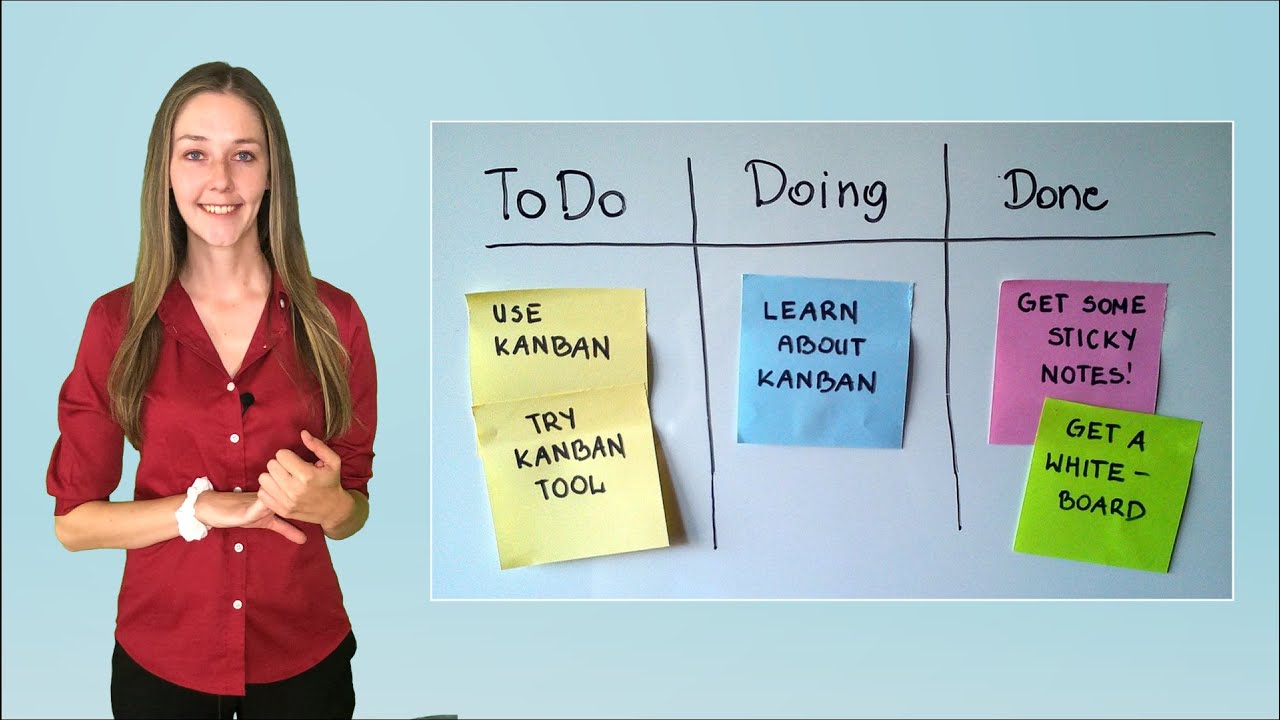The photograph depicts a young woman with sandy blonde hair, dressed in a red burgundy button-up blouse and black pants, standing and smiling at the camera. She is giving a presentation beside a project board divided into three sections titled "To Do," "Doing," and "Done." The board, crafted with one horizontal and two vertical lines, organizes tasks with sticky notes of various colors. Under the "To Do" category, there are two yellow sticky notes that read, "Use Kanban" and "Try Kanban Tool." The "Doing" category features a blue sticky note stating, "Learn about Kanban." In the "Done" section, two purple sticky notes say, "Get some sticky notes," and "Get a white board." The woman is further accessorized with a white scrunchie hair tie around her right wrist. The entire scene is set against a light gray background.